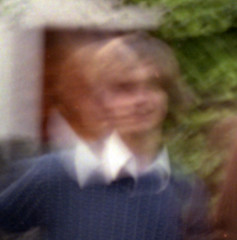The image depicts a young Caucasian man with medium-length, light brown to blonde shaggy hair, parted on the side with sideswept bangs reaching down to a white collared shirt. He is wearing a navy blue, ribbed sweater or cardigan over the white Oxford shirt. The photo is very blurry with a double exposure effect, creating a disjointed, almost ghostly appearance. Despite this, he appears to be slightly smiling. The background features a large green bush or tree to his right, and a dark brown door set against a white building, suggesting the photo was taken outside near a house. There also seems to be some brown shading in the foreground, possibly indicating the presence of another person. No text is present in the image.